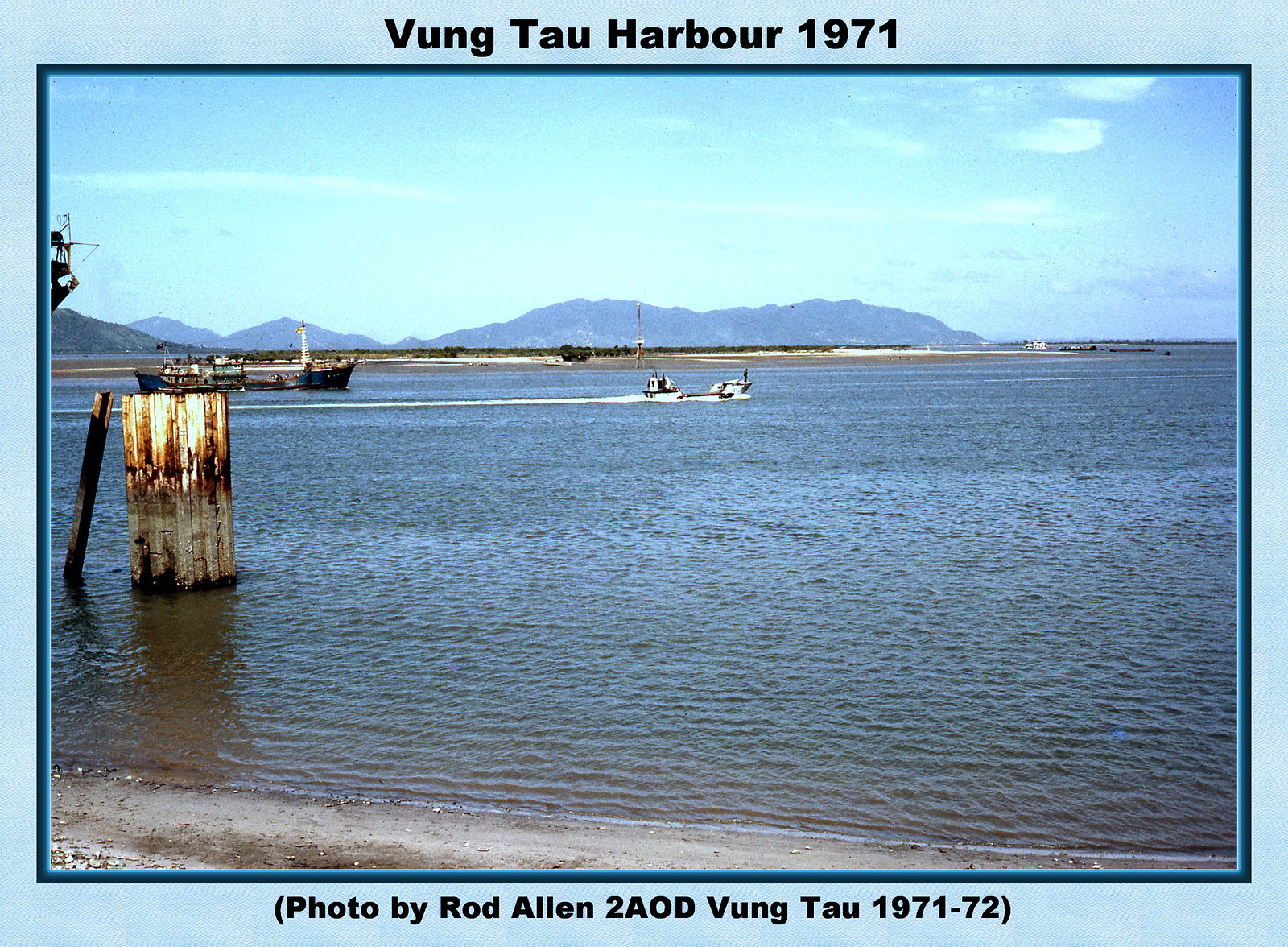This is a scenic photograph with a light blue border and black inner border, reminiscent of a postcard from Vietnam. At the top of the border, the text reads "Vung Tau Harbor 1971," and at the bottom, it says "(photo by Rod Allen, 2AOD, Vung Tau 1971-72)." The image captures a wide, dark brownish body of water with the faint shoreline in the distance. In the foreground to the left, there's a white buoy, and nearby, a rusted white post with another post leaning against it. The scene includes a large vessel on the left and two smaller tugboat-like ships chugging in the center. The background reveals dim mountain ranges and land formations stretching into the water. The overall color palette features a lot of blue tones, from the sky to the water, contrasted by earthy browns and whites.